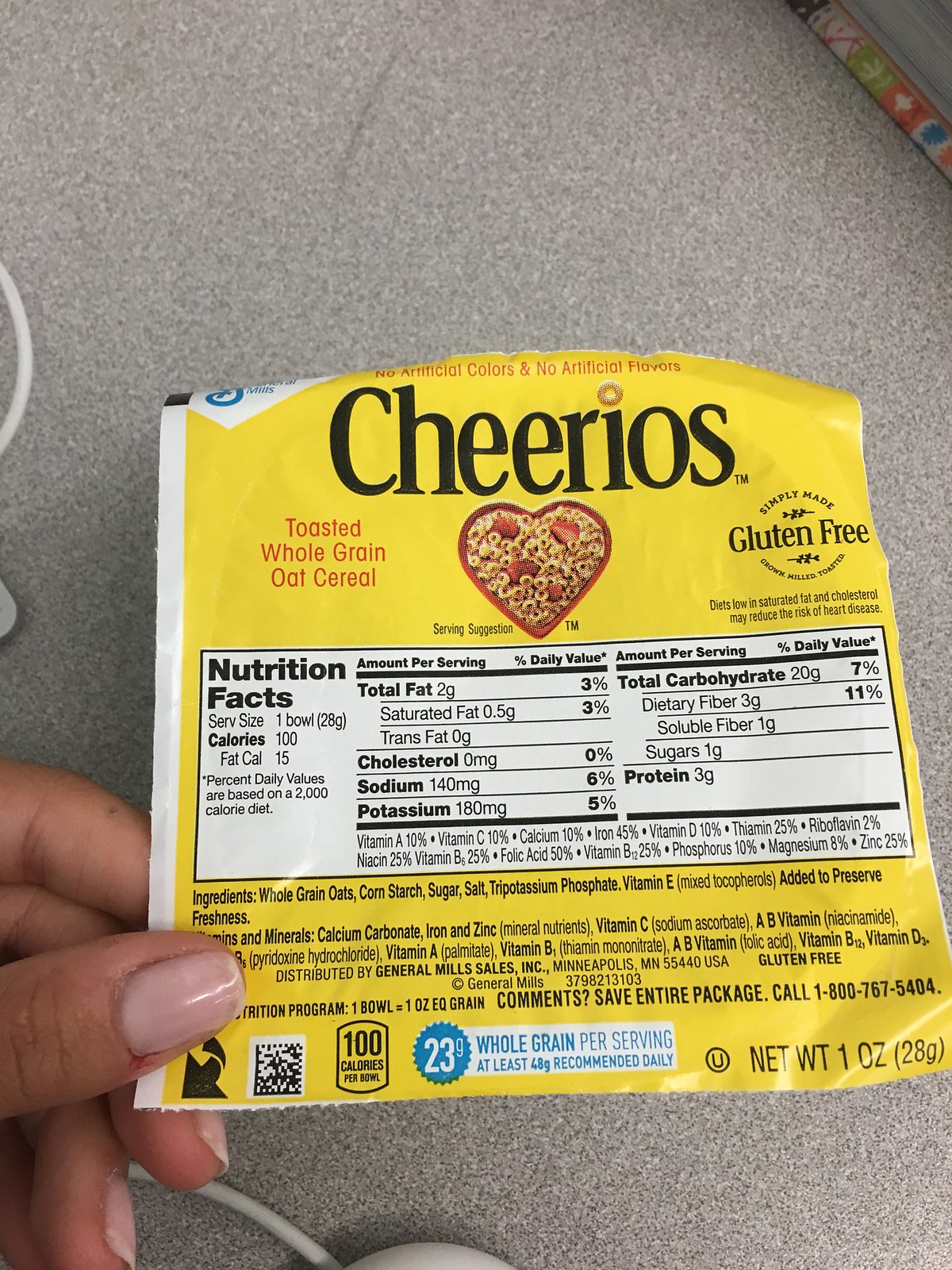This image captures a detailed close-up of a Cheerios cereal box label being held by a person's hand with light-colored polished nails. Set against a predominantly gray background, possibly a computer desk, a mouse is partially visible at the bottom of the frame. The hand appears on the left side, holding up the bright yellow label. Prominently displayed at the top are the words "Cheerios Toasted Whole Grain Oat Cereal" in black letters and "General Mills" in the top left corner. A red heart-shaped bowl in the center contains Cheerios and cut-up strawberries. The label highlights that the product is "Gluten Free" and shows a yellow marker indicating "23g Whole Grain per Serving." Below this, a white rectangular section provides detailed nutritional facts and ingredients. The packaging also indicates a net weight of one ounce at the bottom right.